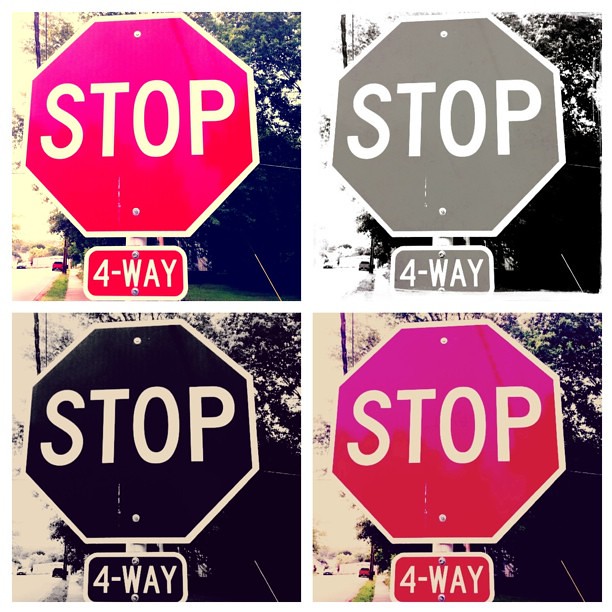The image is a geometrically divided collage featuring four visually altered photographs of the same stop sign and accompanying "four-way" sign in natural light. The collage is arranged in two rows and two columns, with each quadrant depicting the stop sign in a different stylistic treatment. The top left image shows the stop sign in its standard red color and white lettering, illuminated by natural light. The top right quadrant presents the sign in a grayscale format, making the red appear as a light gray against a white background. The bottom left quadrant intensifies the black and white contrast, resulting in a deep black background with stark white lettering. The bottom right image shifts the red hue towards an almost orange shade, giving the stop sign a washed-out appearance. Each photograph retains the classic hexagonal shape and all-caps font typical of American stop signs, emphasizing the contrast in colors and intensity while keeping the central imagery unchanged.